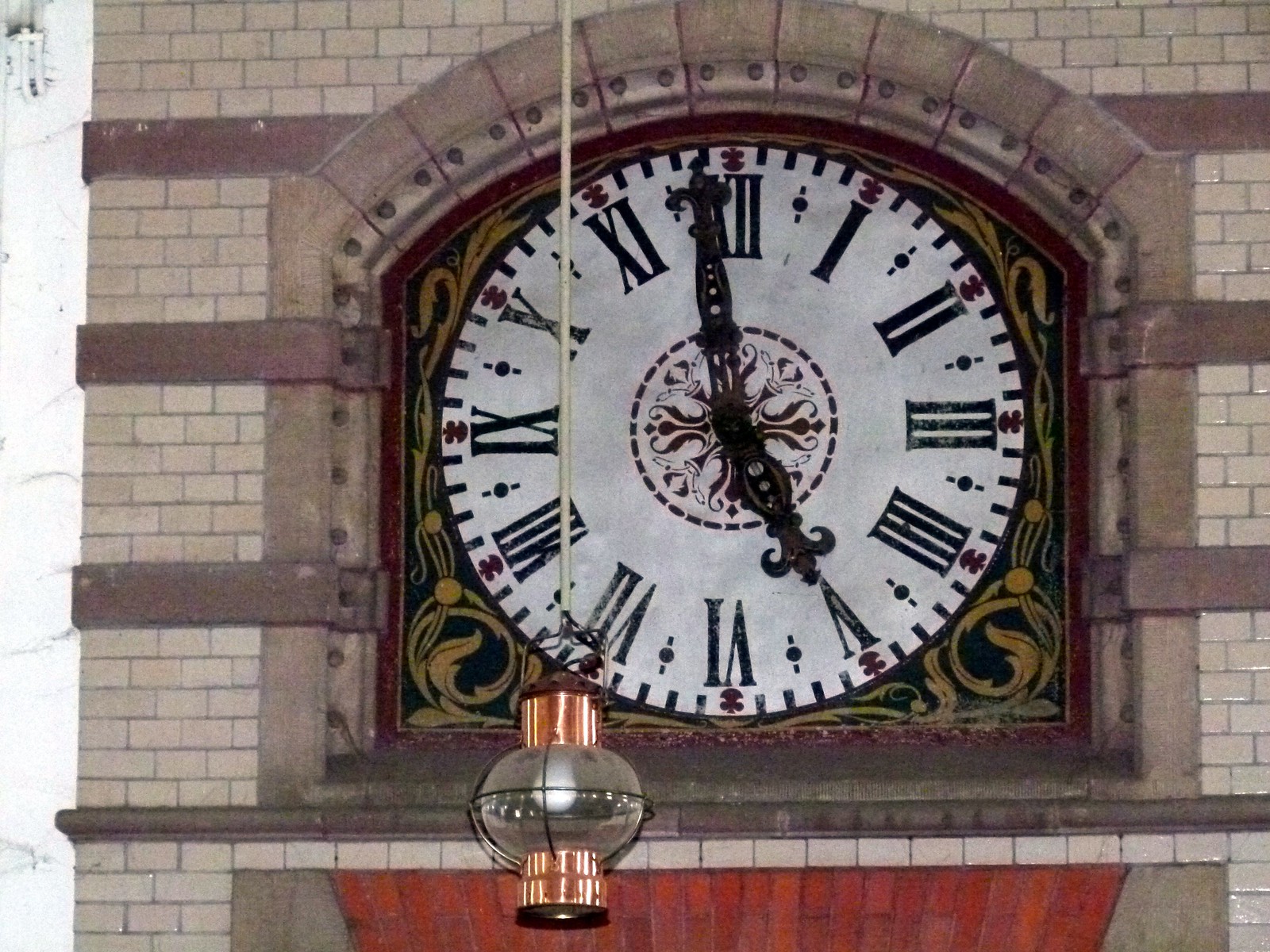This color photograph captures an exterior view of a brick clock tower made of light beige or pinkish bricks. Dominating the upper portion of the image is an ornate, large analog clock framed by a stone archway. The clock face is silverish white and features Roman numerals, with the current time showing a minute before 5 o'clock. The clock's hands are adorned with a fleur-de-lis design, adding to the intricate detail. Surrounding the clock is an outer edge tinged red and embellished with a yellow pattern on a black background. Suspended in front of the clock on a cord is a lantern, which has a glass body with a brass or copper top and bottom, currently unlit. This photograph focuses closely on the clock, the lantern, and this section of the tower, excluding other elements of the building or surroundings.